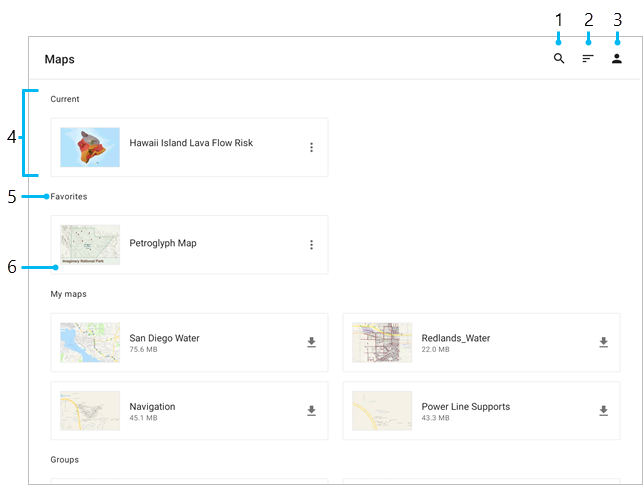This image is a detailed screenshot of a maps feature, seemingly part of a tutorial. The main body of the image, set against a white background, showcases a map interface. In the top-left corner, there’s a prominent label that says "Maps."

Underneath are several subsections. One labeled "Current" displays an image of Hawaii Island with a lava flow risk map. This map is characterized by a deep blue ocean background and a landmass in white, though the intricate details aren’t easily discernible.

Another subsection, labeled "My Maps," lists various maps such as "San Diego Water," "Redlands Water," "Navigation," and "Power Line Supports," indicating an infrastructure focus. Next to each map, there is an option to download, with file sizes noted, such as 75.6 MB and 43.3 MB.

Further down, there is a section titled "Groups." Emerging from the image are several icons, each numbered to indicate their function: 
1. Search function,
2. More options,
3. Person profile,
4. Current section,
5. Favorites section.

Additionally, the "My Maps" section appears again at the bottom, mentioning a "Petroglyph Map" under favorites.

This descriptive caption provides a clear, detailed overview of the map interface and its features, as depicted in the screenshot.